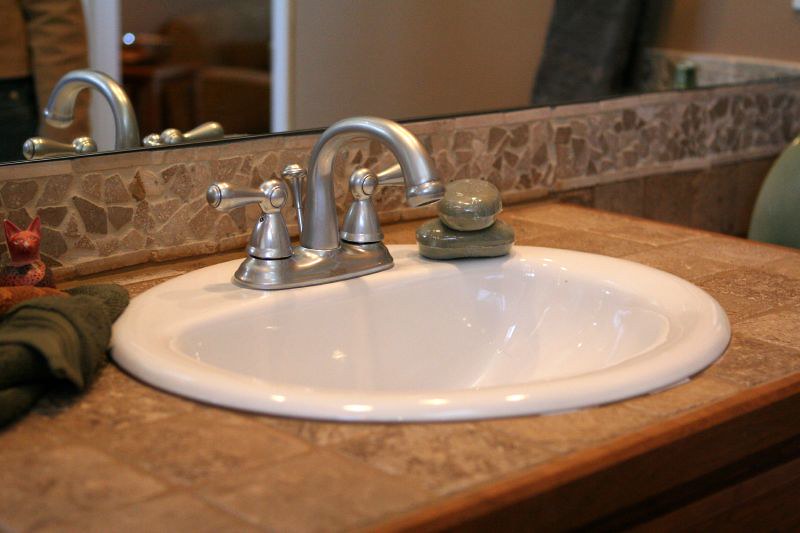A detailed sink setup is showcased in this photograph, featuring a meticulously crafted stone tile countertop that extends from the bottom left up to the right. The countertop is enhanced by a reddish-brown wooden front. Central to this arrangement is a glossy white circular sink, its surface capturing and reflecting white light from various angles. Emerging from the rear of the sink is a sleek, matte metallic faucet, with a curving spout gracefully extending from its base. The faucet is flanked by two taps on either side, each with a rounded, cone-shaped base and a teardrop-shaped handle, oriented in opposite directions—left and right.

To the right of the sink, two stone-like bars of soap are stacked, their glossy texture distinguishing them from actual stones. On the left, an abstract red-headed cat statue adds a whimsical touch, while a folded gray towel is neatly placed nearby. The sink also features a small, thin backsplash made of irregularly shaped stone pieces set within a frame of rectangular stones. Above this arrangement, a bright, reflective mirror captures the top of the faucet, adding to the harmonious balance of the conurbation.